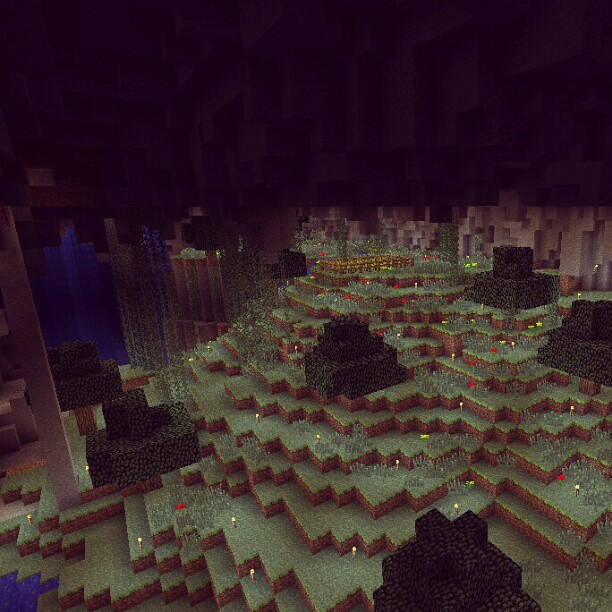This is a vibrant, color image that appears to be a scene from a computer game. The top portion is predominantly black, creating a stark contrast with the vivid detail below. In the central and foreground area, we observe a hill or mountain formed by layers of green-topped blocks with sharp, square jutting edges. These layers cascade down the hill in a zigzag pattern with brown-bordered sides, resembling terraced terrain or possibly a digitally-rendered landscape akin to a stepped bog in County Mayo, Ireland.

Scattered randomly across the terrain are small, luminescent yellow lights, providing an ambient glow that enhances the mysterious atmosphere. Around the base of the hill, there are numerous small piles of black bricks, reminiscent of turf stacks often found in the Irish countryside. Additionally, towards the left side of the image, a few stacks of dark blue bricks punctuate the scene, adding to the array of textures and colors. Overall, the image captures a rich and intricate landscape, blending natural and digital elements in a mesmerizing display.